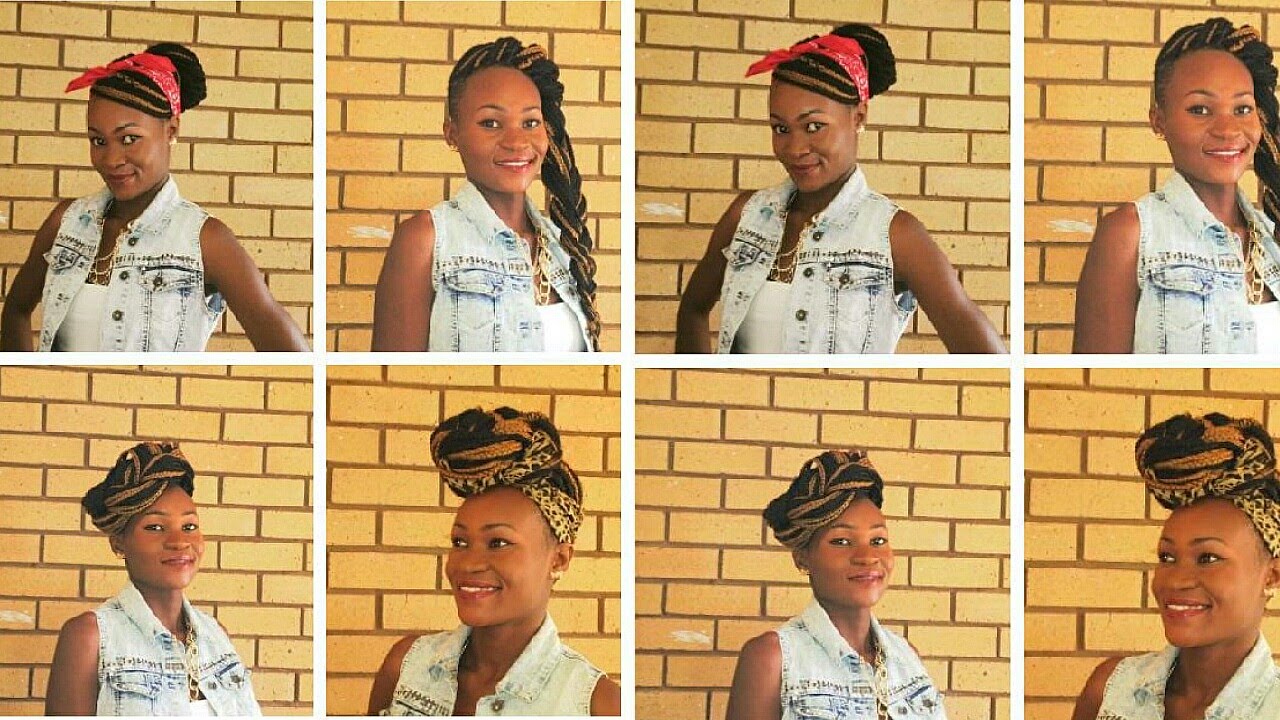The image showcases a set of eight photographs featuring the same young African-American woman, possibly Caribbean, against a yellow brick wall. Each photo highlights different hairstyles, all adorned with long braided extensions incorporating both black and blonde braids. She wears a consistent outfit throughout: a white tank top paired with a sleeveless, stonewashed denim vest with three buttons.

In the top left photo, she artfully coils her hair into a Nefertiti-inspired bun secured with a red bandana. The next photo displays her braids cascading loosely in a side ponytail. Notably, the third and fourth photos are duplicates of the first and second ones, respectively. On the bottom row, the first image mirrors her hair coiled meticulously around her head. Adjacent to it, she gazes in the opposite direction, sporting a leopard-print headband that complements the curled hair on her forehead. The final two photos repeat these hairstyles. The consistent repetition emphasizes her versatile styling while maintaining a visual harmony throughout the set.